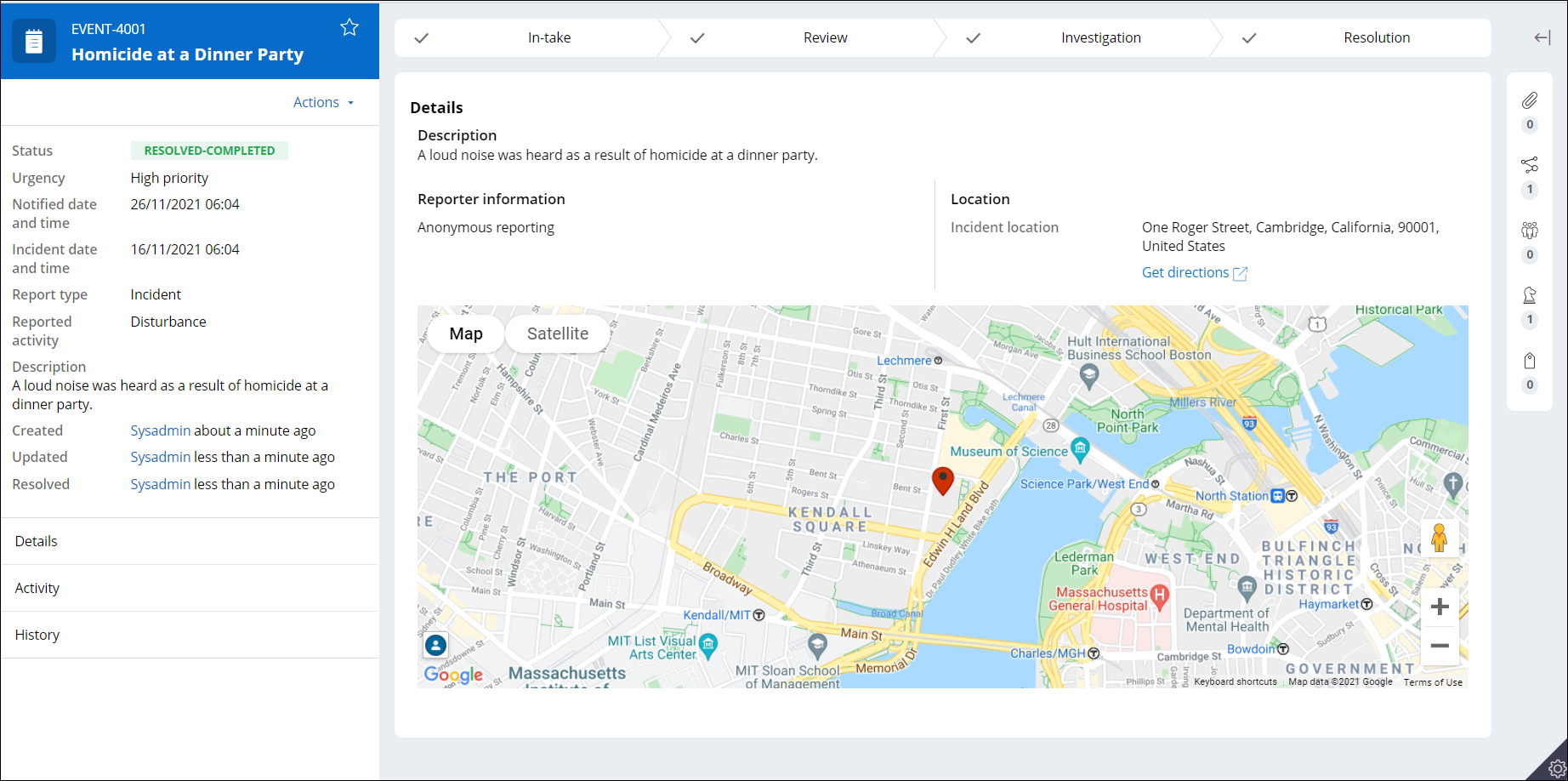A screenshot from an unidentified application, possibly related to law enforcement or crime reporting, shows a detailed log of an event labeled "Homicide at a Dinner Party." The event is listed under ID "4001" twice, with the label highlighted in blue. The left-hand column offers an expandable "Actions" menu and provides comprehensive details about the event.

- **Status:** The incident is marked as "Resolved - Completed" in green.
- **Urgency:** High priority.
- **Notified Date & Time:** Includes precise timestamps.
- **Incident Date & Time:** Provided with exact details.
- **Report Type:** Classified as an "Incident."
- **Reported Activity:** Noted as a "Disturbance."
- **Description:** Details that a loud noise was reported, resulting in a homicide at a dinner party.

The event log chronicles the timeline:

- **Created:** By the user 'sysadmin' approximately one minute ago.
- **Updated:** Less than a minute ago.
- **Resolved:** Less than a minute ago.

Additional sections for "Details," "Activity," and "History" are present but currently empty. The main section of the interface includes a map at the bottom pinpointing the location of the incident. Above the map, further details, descriptions, reporter information, and the incident location are displayed. On the right-hand side, there are options to share the incident report and execute various action items, though their specific functions are not described.